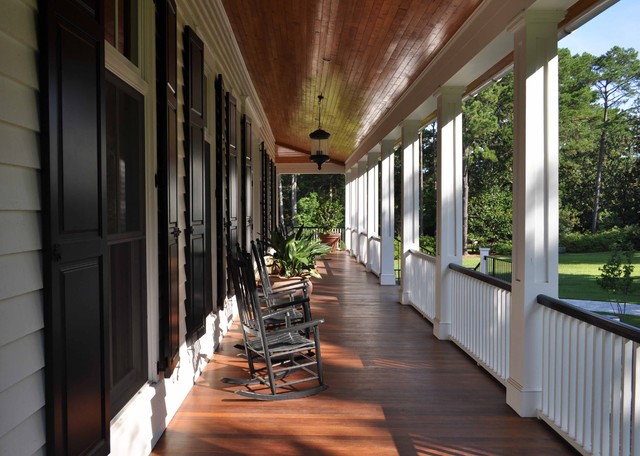This image captures a serene daytime scene of a long, wraparound front porch on a white house with black shutters. The porch, with its wooden ceiling, features a row of black wooden rocking chairs and potted plants that add a touch of greenery. The white railing, topped with a black handrail, is complemented by sturdy white columns supporting the porch's roof. A hanging lamp adds to the charm of the setting. Sunlight streams through the trees in the front yard, casting gentle light across the grassy lawn and enhancing the view of the blue sky. The combination of the comfortable porch seating, lush greenery, and the inviting path leading up to the house creates a picturesque and inviting atmosphere.